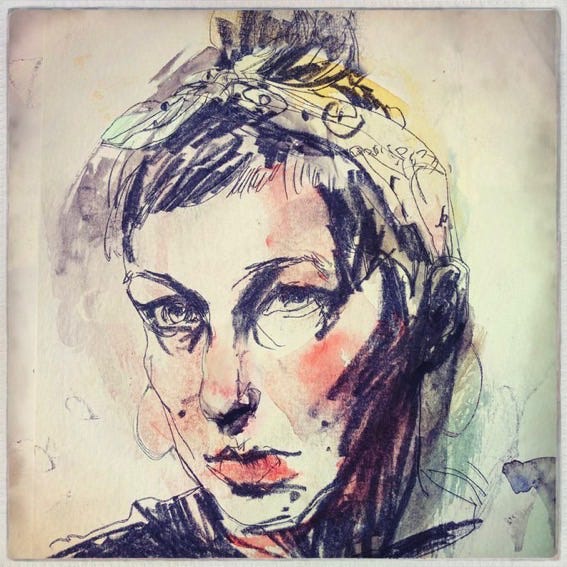The artwork in question is an intricate colored pencil sketch, heavily rendered with a black pencil, portraying a woman gazing to the left. She sports a short hairstyle, partially gathered into a ponytail and secured with a headband adorned with musical notes, which doubles as a yellow scarf wrapped through her hair. Her bangs frame a large forehead, and she has thin eyebrows, almond-shaped eyes, a thin nose, and red lips. There are pinkish hues on her cheeks, suggesting either artistic blushing or shadowing. Her hair, cropped just above her ears, might be accompanied by moles or ink splashes, adding to the textured, somewhat messy style of the piece. The use of various colors, including black, pink, red, blue, and yellow, accentuates the character's features and the atmospheric shading, with light casting shadows from above. There's a vague background presence, potentially including a dog, further complicating the scene's narrative depth.